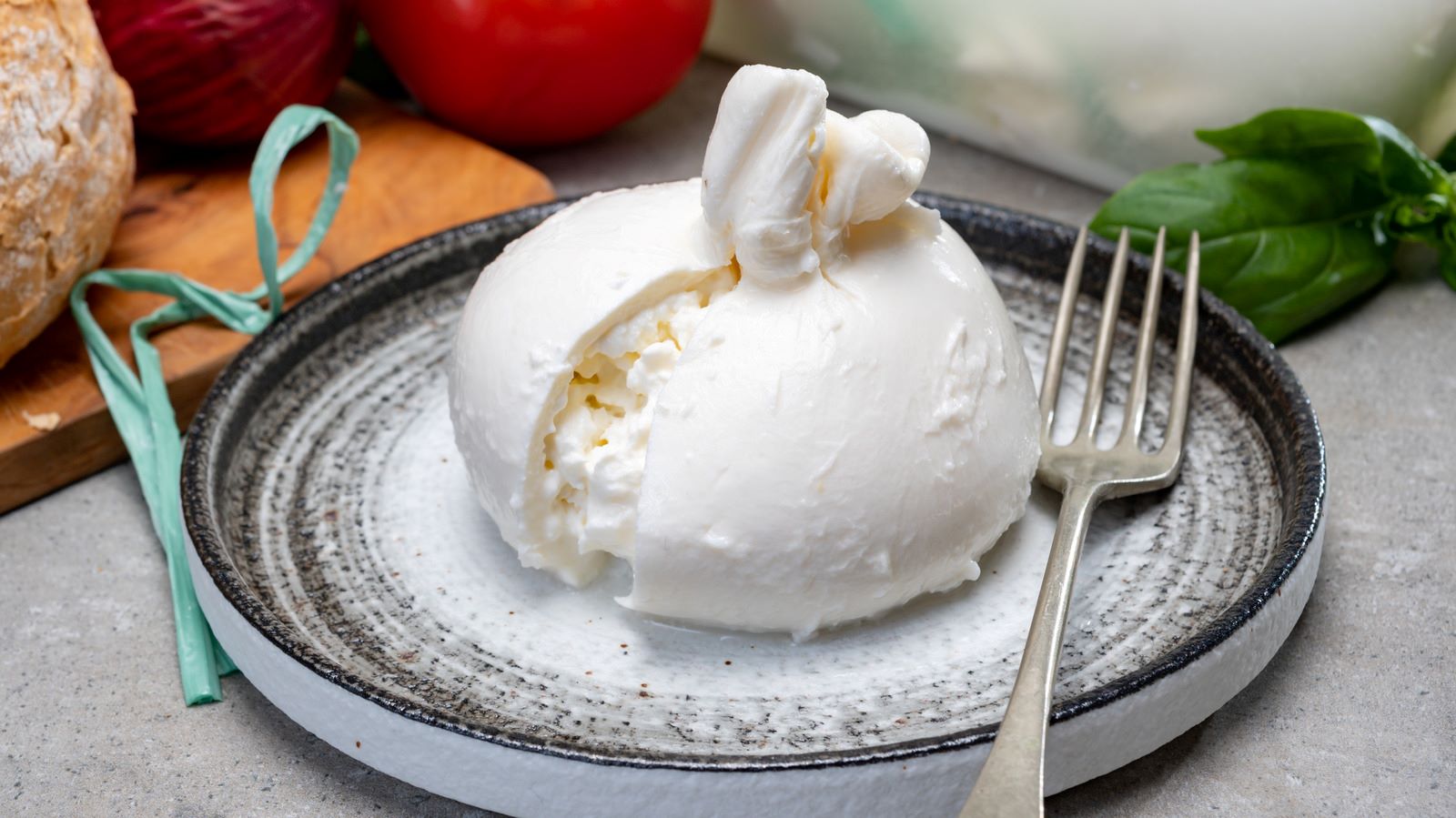The image features a shallow silver plate with a distinct black rim, placed on a gray countertop. A silver fork rests on the plate, which holds a soft, creamy dessert resembling a white round mound that has been split open to reveal a cottage cheese-like substance inside. To the right of the plate, a sprig of parsley is visible. In the upper left-hand corner of the background, a brown cutting board holds a tomato and an onion, possibly accompanied by some bread. A green ribbon made of natural fibers ties around these items, adding a rustic touch to the scene. The detailed textures and elements provide a rich, inviting culinary setting.